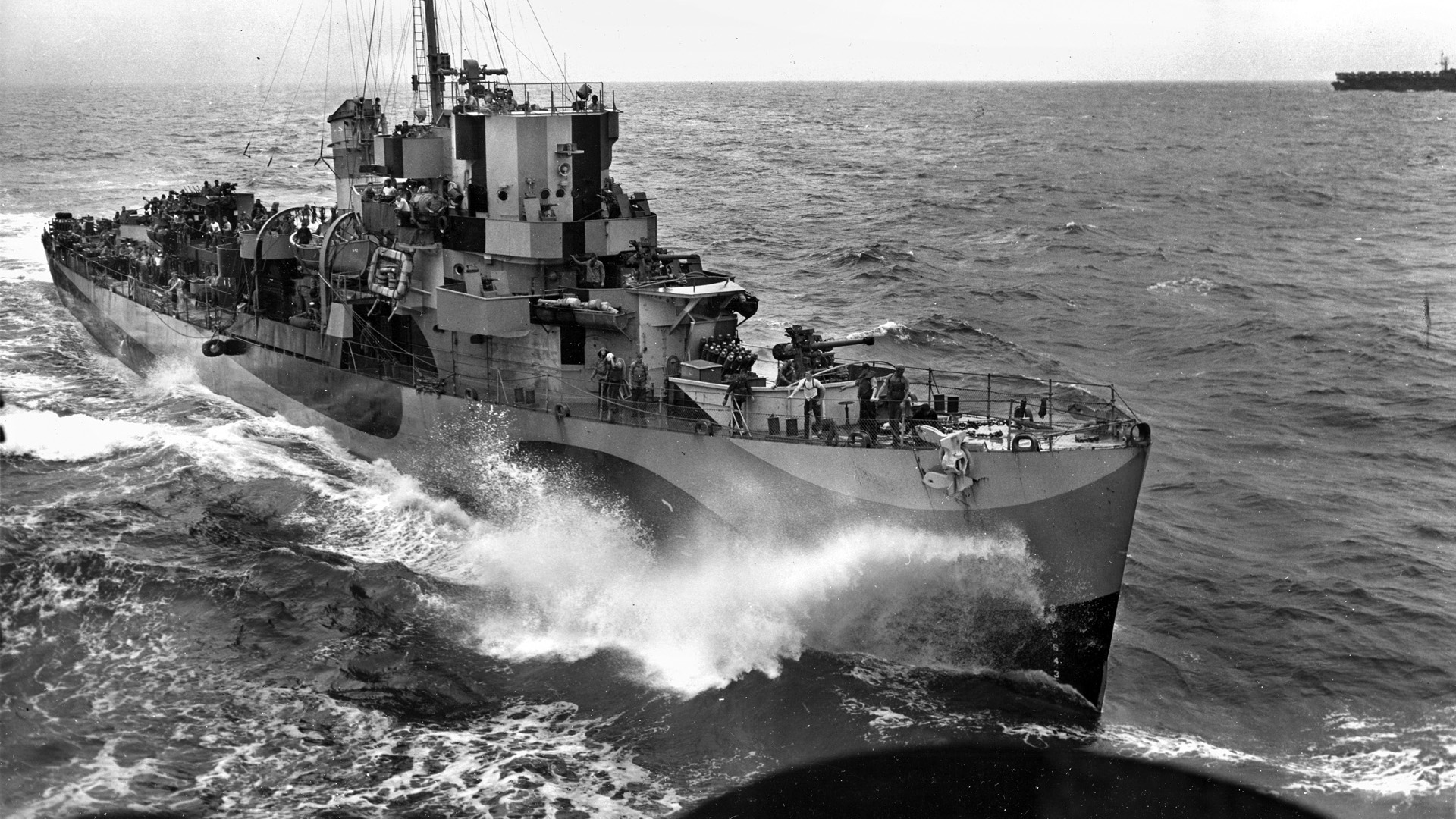The black and white photograph captures a large naval battleship cruising through the ocean, evidenced by the frothy waves crashing along its hull. The horizon line where the water meets the sky stretches across the top of the image, framing the scene under what appears to be overcast weather. The ship, unmistakably a military vessel due to a massive mounted gun towards the front, is teeming with numerous sailors, notably gathered at the rails both in the front and rear sections of the deck. Some men are shown leaning over the rails, while others are looking directly at the camera, suggesting the photo was taken from nearby, potentially another vessel, a drone, or an aircraft. The ship, with its high stacked center and rigging devoid of sails, indicates a motorized propulsion system. Additionally, the vessel's grey tones and bustling activity of sailors emphatically reinforce its military purpose. In the far background, just at the edge of the upper right corner, part of another ship is faintly visible, pointing to a fleet or convoy setting. The dynamic motion of the ship, accentuated by the bobbing and dancing in the water, underlines the lively and vigilant scene captured in this historic marine snapshot.